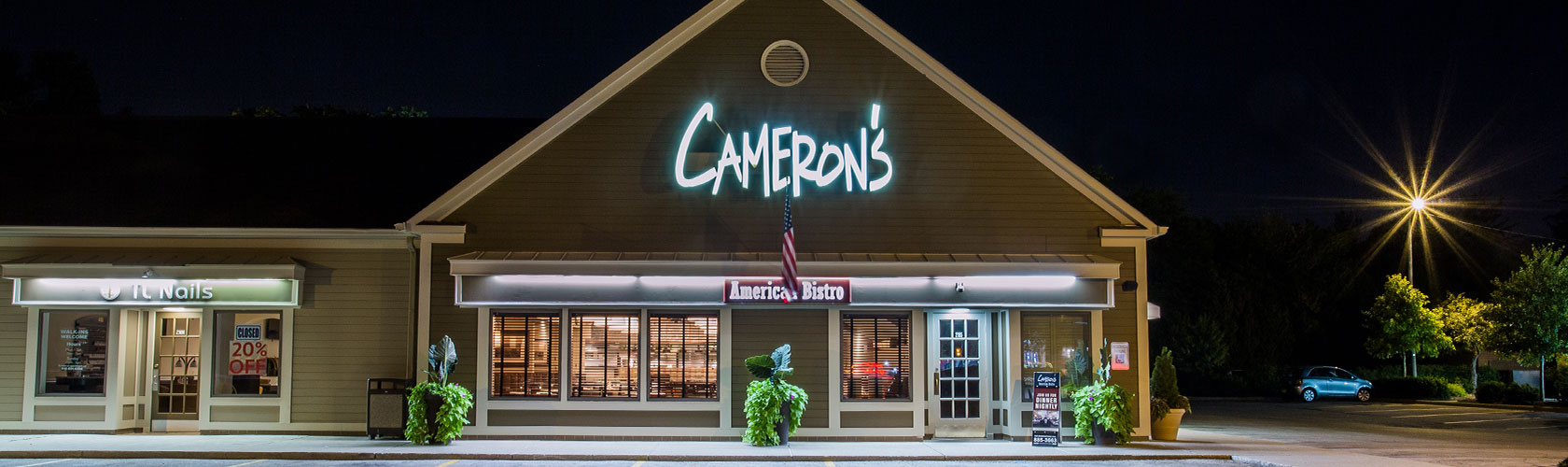The image depicts the front facade of a restaurant named Cameron's during nighttime, likely a high-resolution digital creation. The building features a pointed, upside-down V-shaped roof. "Cameron's" is prominently displayed at the top center in white text, with a larger "C" lining up with the sign's apostrophe. Below, a red sign reads "American Bistro" in white text, sitting below an American flag projecting upwards. The interior and exterior are well-lit, enhancing the ambiance. To the left of Cameron's, a nail salon with a sign that reads "20% off" in red text, possibly named "See Nails" or "IT Nails," shares the building. Bushes adorn the front, and a blue compact car, possibly a Prius, is parked in the lot to the right. Visible above the scene are green trees and a streetlight.